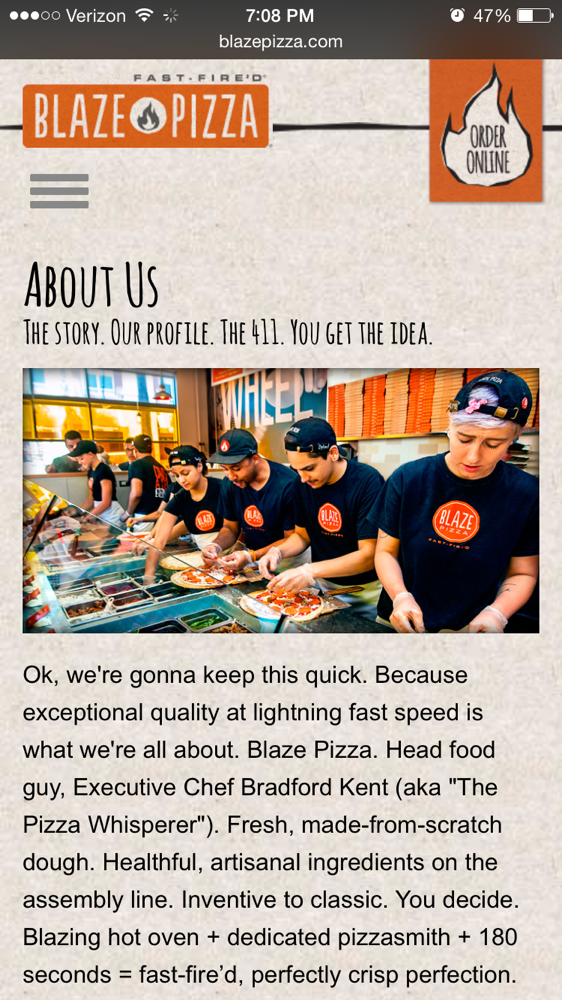The screenshot shows a mobile phone interface with Verizon's service indicator at the top, displaying "3 out of 5" bars and the time "7:08 PM" with a 47% battery life remaining. The user is browsing the Blaze Pizza website, indicated by the prominent Blaze Pizza logo on an orange background with a fire symbol and the words "Order Online" inside the flame. The background is a soft tan color, complementing the website's aesthetic.

To the right of the logo, there is an option to explore more about Blaze Pizza with a hamburger menu icon, offering the "About Us" section. In this section, the company's story is highlighted with a picture of an assembly line where pizzas are being made. The caption notes that Blaze Pizza prides itself on exceptional quality and speed, emphasizing their fresh, made-from-scratch dough, and artisanal ingredients. Executive Chef Bradford Kent, known as the Pizza Whisperer, assures customers of their inventive to classic pizza options cooked in a blazing hot oven by dedicated pizza smiths within 180 seconds, delivering a perfectly crisp pizza.

The clear and detailed focus of the screenshot is on the swift and quality-driven pizza-making process offered by Blaze Pizza, inviting the viewer to experience their fast-fired, artisan pizzas.